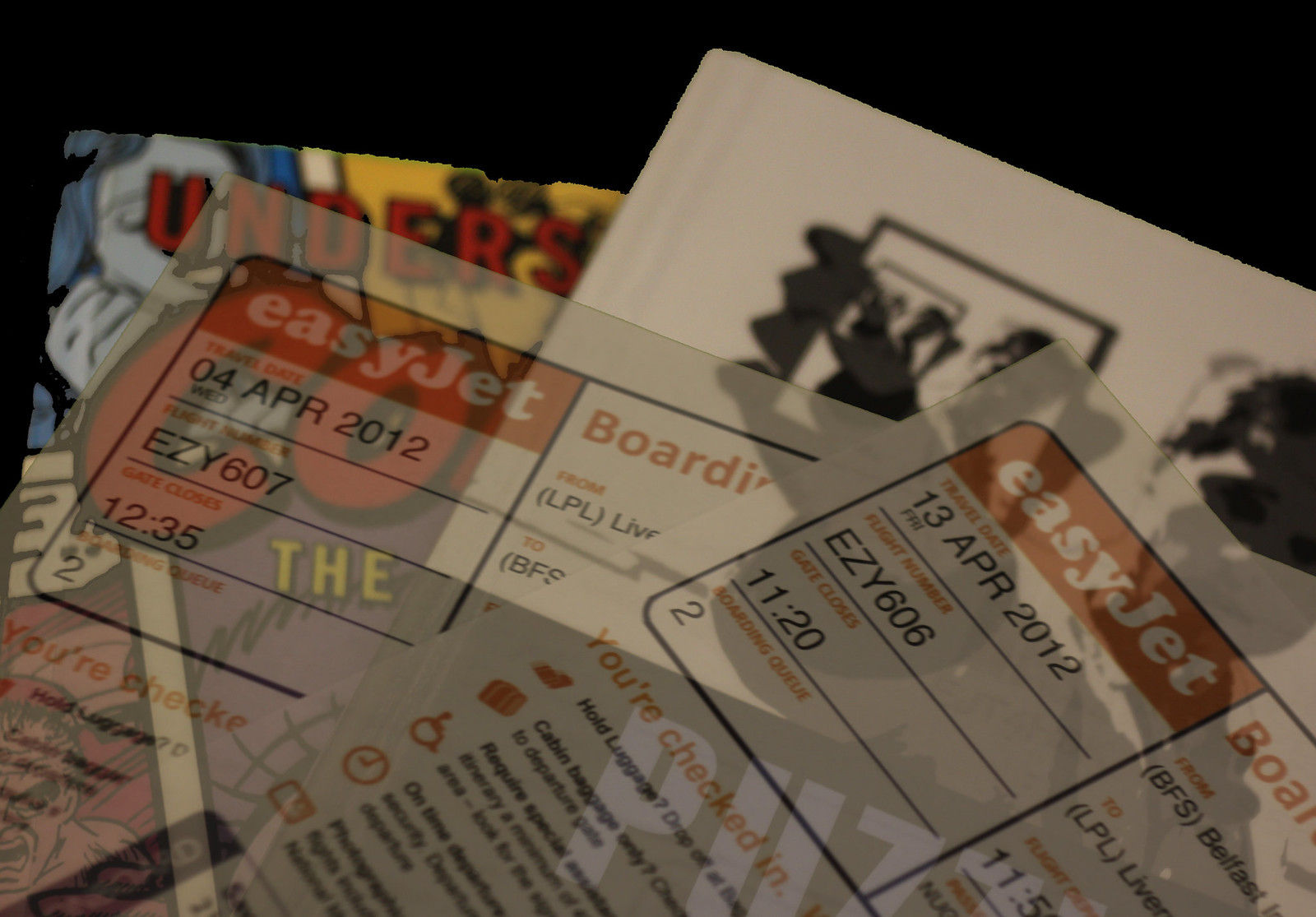The image showcases a collection of overlaid documents against a black background, which is visible around the edges. In the upper left corner, there's the partial image of a comic book, featuring a woman with blue hair holding a phone and the red lettering "UNDERS". Beside and partially covering the comic book is a white page displaying black images. Prominently overlaying these is a red and white EasyJet boarding pass labeled "BOARDING" with details including "04-APR-2012", flight number "EZY-607", and time "12:35". To the right, another scattered EasyJet boarding pass, dated "13-APR-2012" with the flight time "11:20", is also visible. The words "THE" in gold lettering and other indistinct large red letters further add to the layered visual elements.